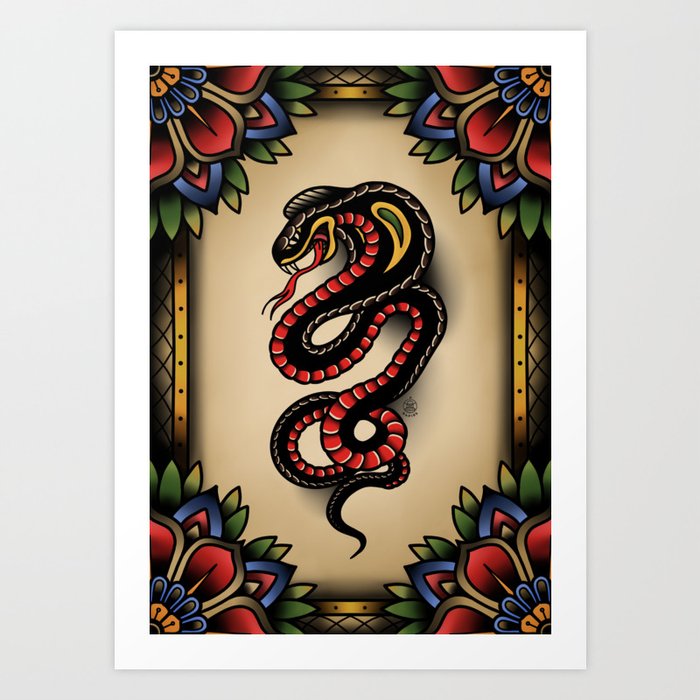This detailed piece of computer-generated artwork depicts a colorful, coiled serpent at its center, set against a tan background. The central image is framed within a vertically aligned rectangular picture with a thick white border, all placed on a solid light gray wall, giving the appearance of a framed painting. The serpent, possibly a cobra, exhibits a striking design with predominant black, red, and gold trims. Its menacing presence is accentuated by its two prominent fangs, a long red tongue with pronged ends, and intricate green and yellow patterns around its hood. Surrounding the serpent, large floral decorations adorn each corner of the frame. These motifs incorporate vivid greens, reds, blues, yellows, and copper hues, adding a rich and vibrant contrast to the overall composition. The golden rail-like adornments on the left and right sides of the frame further enhance its elegant and emblematic appearance, suggesting that the artwork could serve as a logo or crest for a society.